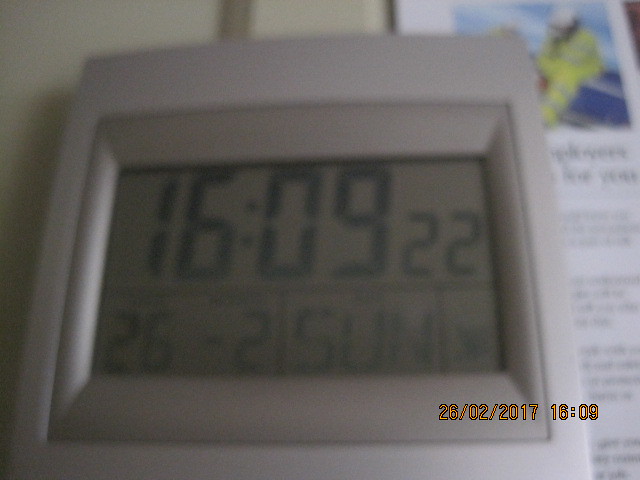The photograph captures an up-close view of a square, off-white digital clock with a thick border. The clock's display has a tan background with black digital numbers showing the time as 16:09:22, translating to 4:09 PM and 22 seconds in 24-hour format. The display is detailed with faint black lines dividing sections. Below the time, the date "26-2" is visible, alongside the abbreviation "SUN" for Sunday, and an indistinct symbol. The bottom of the image features a timestamp in yellow, reading "26-02-2017 16:09." The background is split between a beige wall on the left and a partially visible rectangular white sheet of paper on the right, potentially a book page or brochure, with a yellow and blue image at the top and black text beneath. The bottom right corner of the image is slightly blurry.